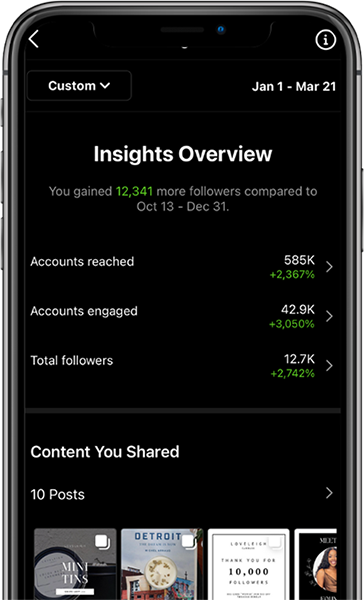The image depicts a sleek smartphone with a reflective silver border, highlighting its modern design. The screen's background is black. At the top of the screen, a white left-pointing arrow is positioned on the left side, while a circle containing a lowercase 'i' is located on the right side. Below this, on the left side, there's a dropdown menu labeled "custom," accompanied by a downward-pointing arrow. Adjacent to this, on the right side, the date range "January 1st to March 21st" is displayed. 

A light gray horizontal line spans the screen, below which, centered, are the words "Insight Overview" in white text. Further below, gray text informs the viewer that they gained 12,341 more followers compared to the period from October 13th to December 31st, with the number "12,341" highlighted in green. Additional spacing leads to more statistics: "Accounts reached 585k" in white text, followed by a right-pointing arrow. Below this, the green text reads "+2,367%". Continuing down, "Accounts engaged" is noted in white text as "42.9k," with another green percentage increase of "3,050%" indicated below.